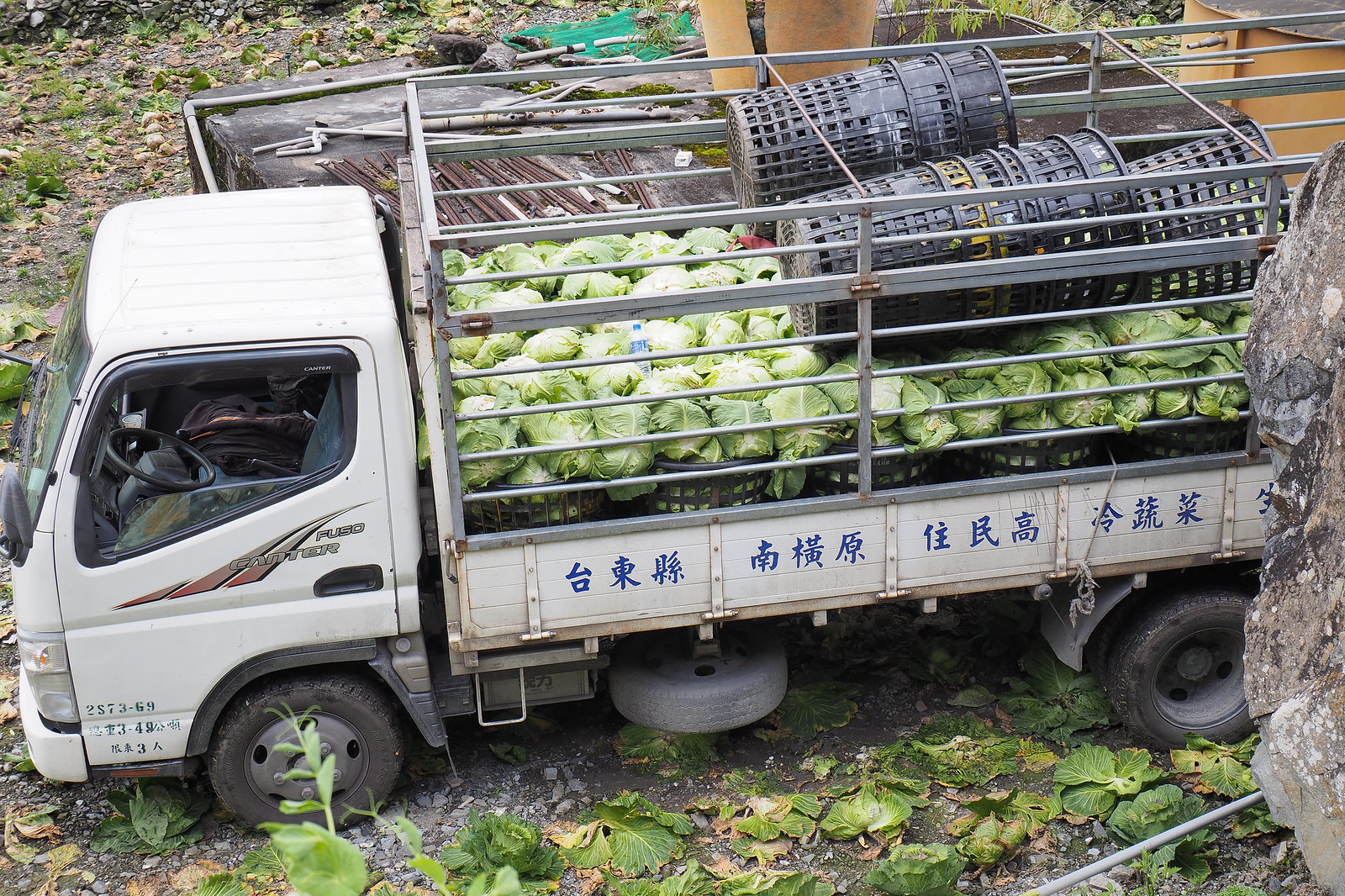In this detailed outdoor scene, a white flatbed truck dominates the landscape, situated in what appears to be a recently harvested cabbage field, with green foliage and scattered cabbage leaves adorning the ground. The truck, which features a large, semi-truck style cab with Asian characters inscribed in blue along its sides, showcases a wooden-walled storage area behind the cab. This storage area is protected by a gray metal fence with hinge points, possibly allowing for side access. The flatbed of the truck is brimming with freshly picked green cabbages, accompanied by several black, plastic, mesh-like baskets presumably used for sorting and washing the vegetables. In the background, two large, orangish-brown containers are visible, though their purpose remains unclear.